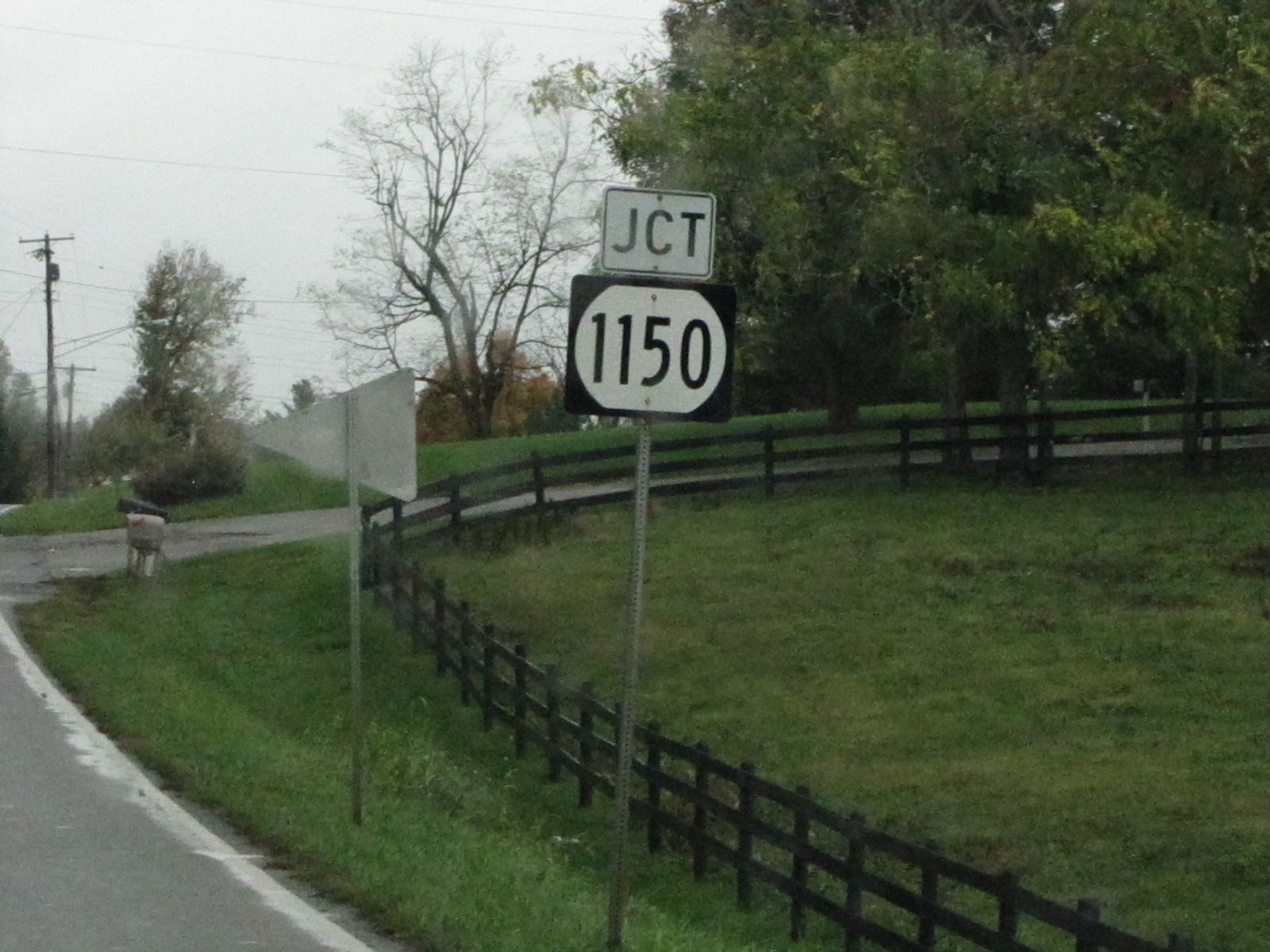The image depicts a rural roadside scene dominated by a prominent road sign indicating "JCT 1150" in bold black letters against a white background. This sign stands tall on a single pole beside a small, seemingly quiet road. Immediately adjacent to it, the back of another road sign faces the opposite direction, revealing only its metallic construction. The setting is complemented by a painted white line running parallel to the road, designed to prevent vehicles from veering into the grass.

In the foreground, a couple of mailboxes—a white one and a black one—stand at the roadside. The scene extends to a brown wooden fence, crafted in a circular pattern around a well-maintained corner lot. This lot, likely part of a residential property or a farm, features lush green grass and several mature trees, enhancing its idyllic quality. Electric poles are also visible, hinting at the infrastructure supporting this rural area. The overall impression is one of tranquility, with clear indications of both natural beauty and human presence.